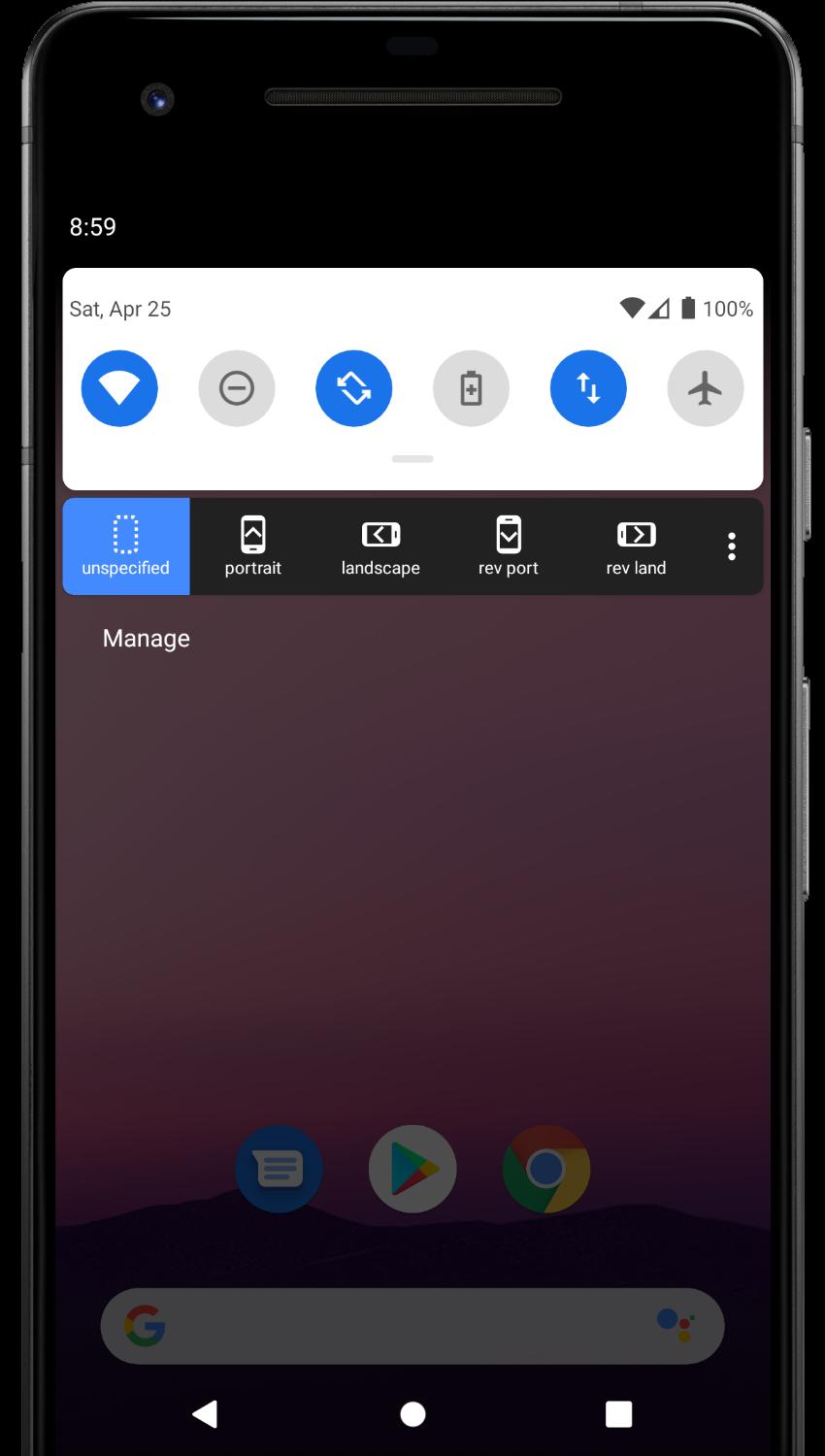The image depicts a mobile phone, which has been photographed, showing the distinct edges and contours of the device. The top portion of the phone is obscured by a black area, but the long, thin speaker is clearly visible, suggesting that this model is somewhat outdated.

At the top of the phone's screen, the time is displayed as 8:59. Below the time, there is a horizontal white rectangle. The rectangle has a shorter height compared to its length, and within it, the first visible line reads "SAT, APR 25." To the right of this line, several icons are displayed: the WiFi symbol, signal strength icon, and a battery indicator showing 100%.

Further down, the screen features a set of circular icons. The first is a blue circle with a white strength icon inside. Next is a gray circle containing another circle with a diagonal line through it. Following this is another blue circle with an icon resembling arrows forming a rectangle, indicating auto-rotation. Adjacent to this is a gray circle with the battery percentage, another blue circle with an arrow pointing up and another pointing down, and finally, a circle with an airplane icon, suggesting flight mode.

At the bottom of the screen, the Google search bar is prominently displayed alongside the icons for text messaging, Google Play, and Google Chrome.